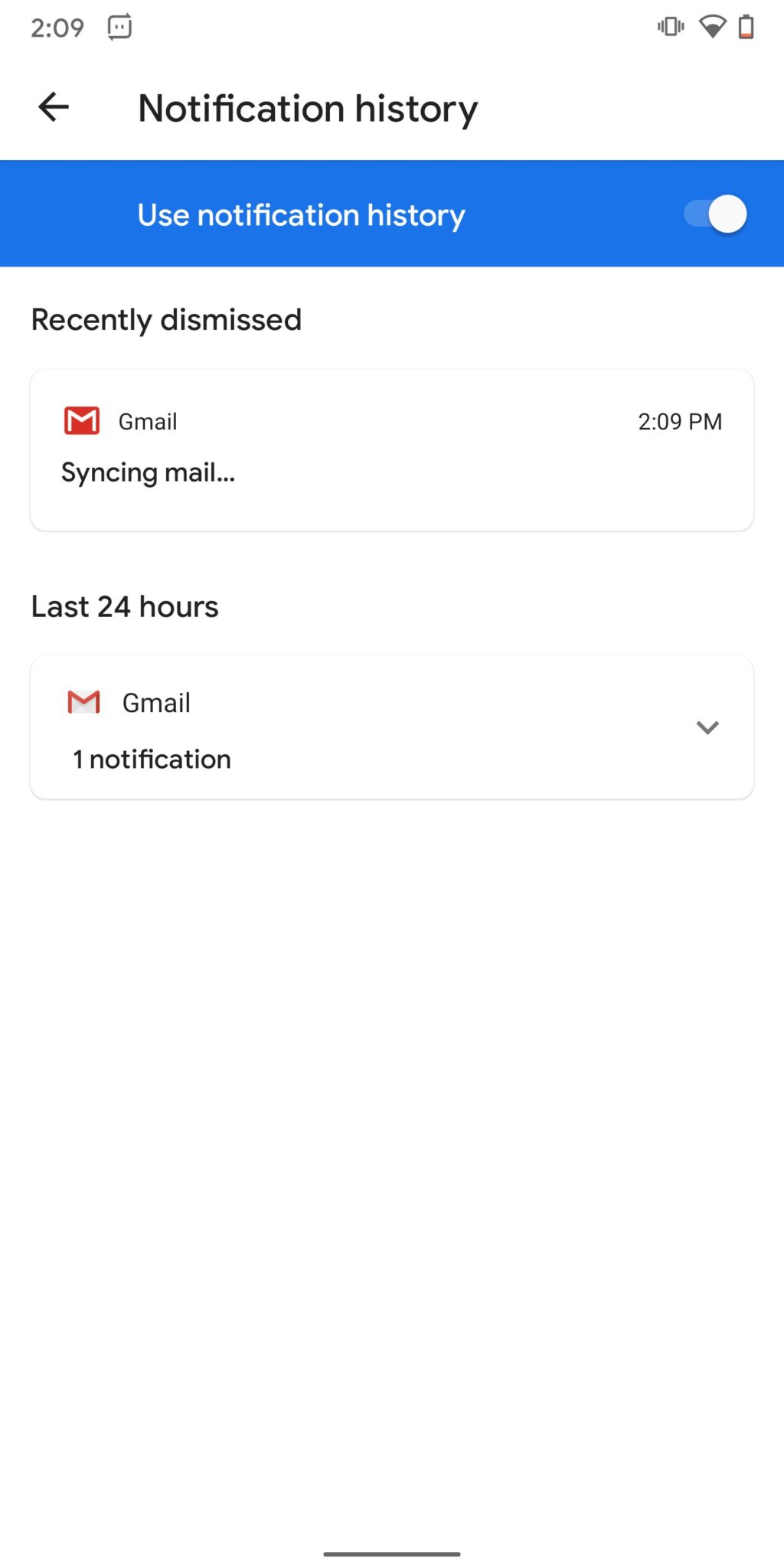This image showcases the screen of a mobile device within an app. The app screen itself has a clean, white background. At the bottom of the screen is a swipe-up bar, indicating the viewer's ability to navigate upwards within the interface.

At the top of the screen, the status bar displays several key elements. On the left, the time reads 2:09, adjacent to an icon resembling a square with two dots inside it. On the right side, icons indicate that the phone is set to vibrate, connected to Wi-Fi, and has a battery that is nearly depleted.

Just below the status bar, a back arrow is positioned to the left of the text "Notification History." Directly beneath this, in bold blue text, is "Use notification history," highlighted with a blue box indicating that this feature is currently enabled.

Further down, under the "Recently dismissed" section, a white box shows that an email app (Gmail) had a syncing mail notification at 2:09 PM. Lastly, under the "Last 24 hours" section, there is another white box indicating that Gmail had one notification. A small dropdown icon appears to the right of this information, suggesting additional details can be revealed.